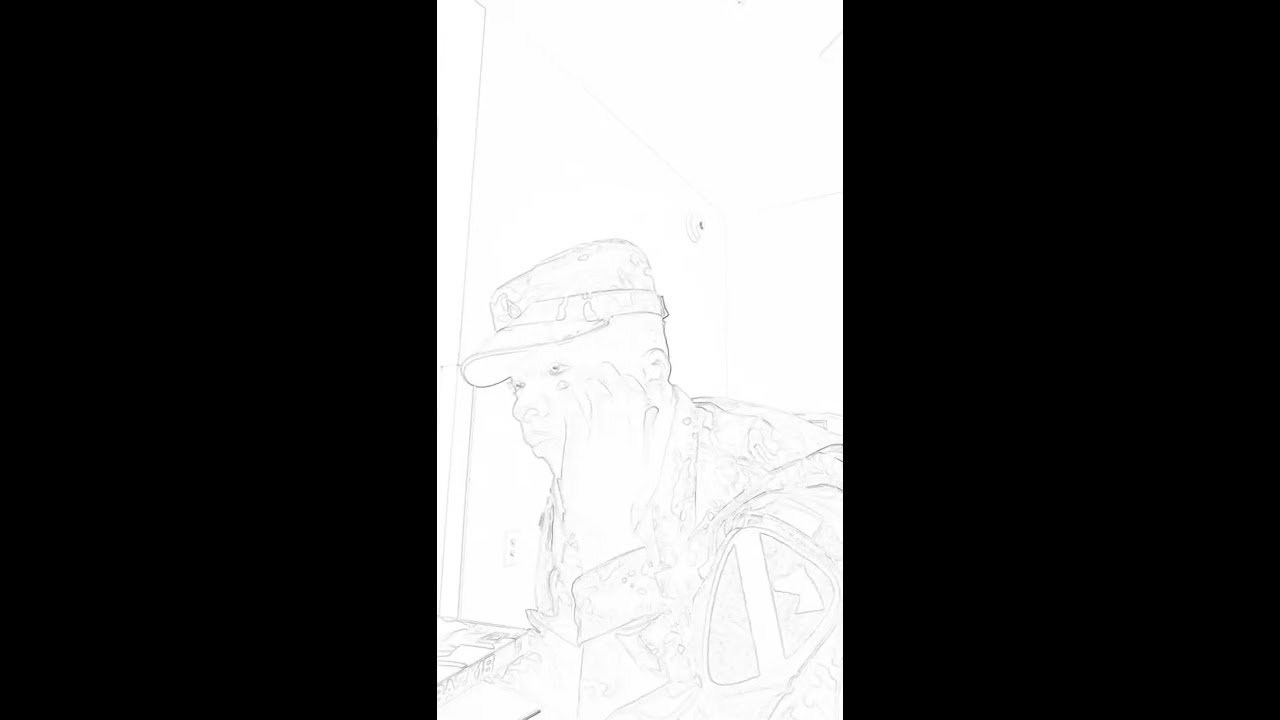The animated slide displays a stark and minimalist image. Dominating the right and left sides are large black vertical rectangles, creating a strong contrast against the entirely white central section. Centered within this white space is an image of a man, either hand-drawn or made to look as such through a filter effect. The man's likeness, depicted in varying shades of gray and faint blue lines, portrays him with his head resting on his hand, gazing slightly to the left. He is dressed in a military uniform, complete with a military-style cap and a patch on his fatigues. The background is devoid of any text or additional objects, heightening the sense of emptiness and focus on the solitary, introspective figure.